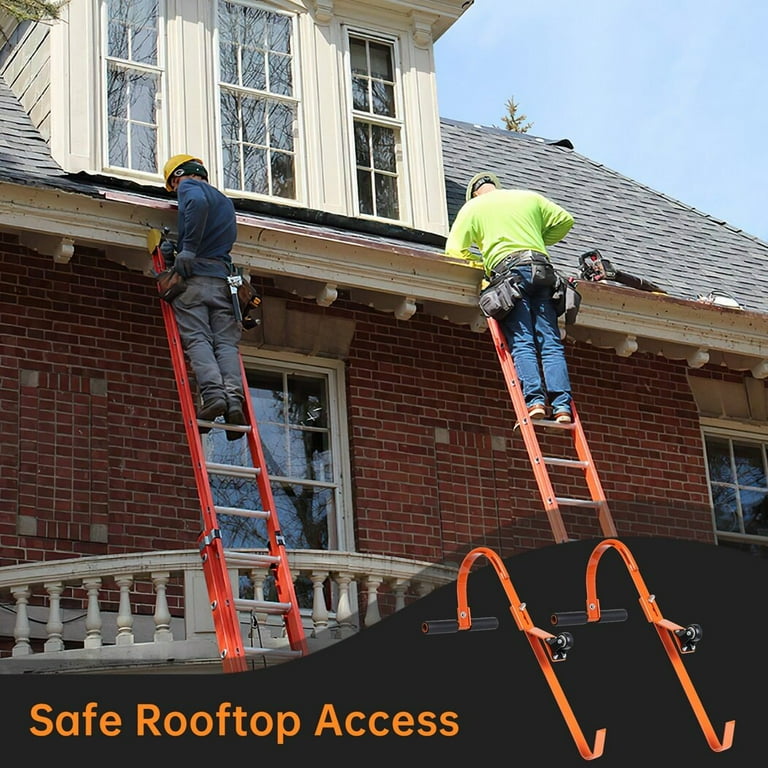This realistic square-shaped photograph taken outdoors during the daytime features two men working on the roof of a red brick house. The house has white windows, a white masonry balcony located below the men, and an exposed white dormer window protruding from a gray roof. The men, standing on orange ladders at the gutter area, are both clad in safety gear, including yellow helmets and work outfits. The man on the left is wearing a blue shirt and gray pants, while the man on the right is dressed in a bright green shirt and blue jeans, both equipped with various tools hanging from their waists. The sky above them is a clear light blue. 

At the bottom of the image, a black swoop with orange text reads "Safe Rooftop Access," accompanied by an image on the right of orange contraptions that appear to secure the ladders to the roof. Additionally, a leaf blower can be seen resting on the roof, highlighting the ongoing construction work. The men are positioned approximately six feet apart, viewed from the back, diligently working to ensure safe roof access.